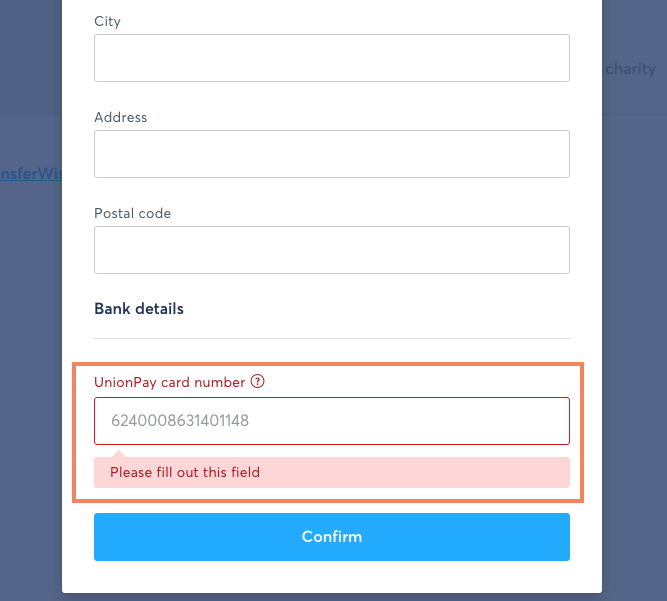In the image, there is a white and blue form designed for collecting information. The form's layout is structured primarily on the left-hand side with several labeled fields. At the top, there is a section labeled "City" with an empty bar intended for the user to input the city name. Directly below, there is a section for "Address," accompanied by a space for inputting the user's address. Following this, there is a field for the "Postal Code," which also features an empty space for entering the postal code.

Further down, there is a section titled "Bank Details" that precedes a horizontal line. Beneath this line is the "Union Card Number" section, where the label and the text are prominently highlighted in red. This section also includes a designated space for entering the numeric details of the union card number.

Additionally, there is a red alert message that reads, "Please fill out this field," indicating mandatory information. At the bottom of the form is a blue-highlighted button labeled "Confirm," which suggests finalizing the form submission.